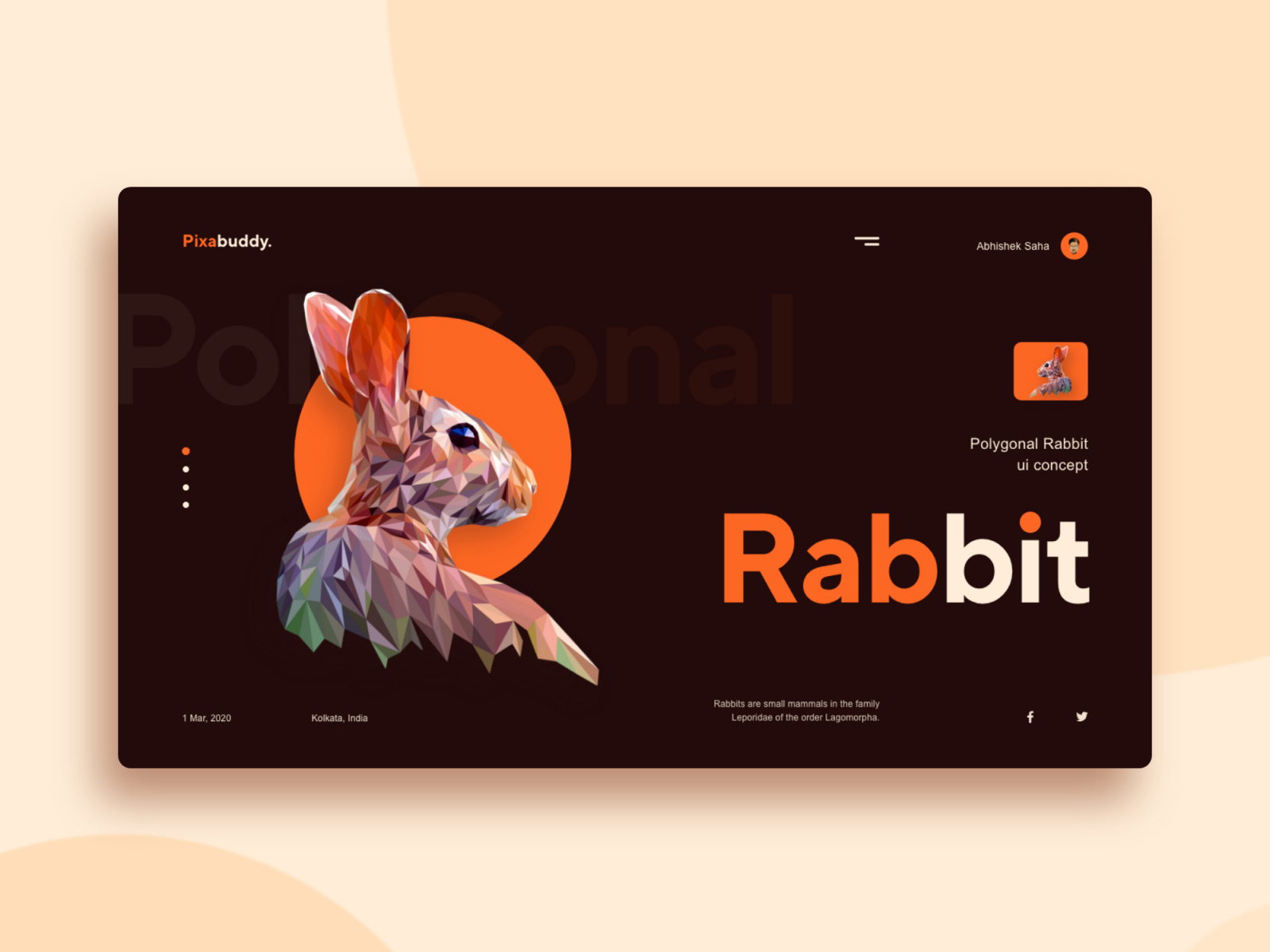The image is a screenshot of a computer screen featuring a design with an off-white background. In the bottom left corner, a light orange circle peeks into view. Another larger light orange circle dominates from the top right, extending toward the center of the screen. In the upper left quadrant, a prominent black rectangle is displayed, showcasing the text "PIXA Buddy" with "PIXA" in orange and "Buddy" in white.

Adjacent to the right of this rectangle, there is a small circular icon with the image of a male figure. Accompanying this icon is a name in tiny font, which appears to be something like "Afgan Safu," resembling an Iraqi name.

Additionally, a large orange circle is positioned toward the left side of the image. In front of this circle, a stylized bunny is depicted, facing right with its ears perked up. The bunny's body consists of geometric shapes resembling diamonds, with a notable black eye. To the right of the bunny, the word "Rabbit" is written, with "RAB" in orange and "BIT" in white, and the dot over the "i" in orange.